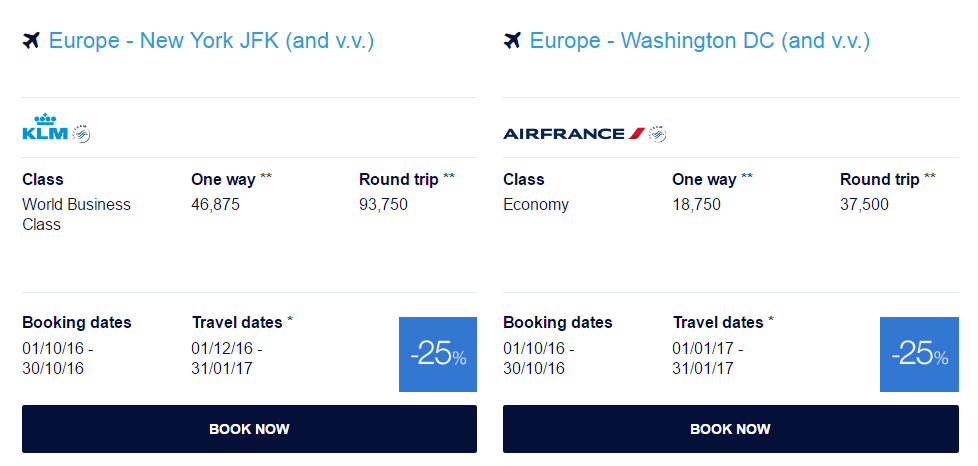This is a screenshot from a travel booking website displaying flight options from Europe to New York (JFK) and Washington, D.C. On the left, the flight from Europe to New York (JFK) is operated by KLM, showcased with their logo. The flight offers World Business Class, with a one-way fare of $46,875 and a round-trip fare of $93,750. The booking dates for this flight are from October 1, 2016, to October 30, 2016, while the travel dates range from January 12, 2016, to January 31, 2017, covering nearly a month's duration.

On the right, the flight from Europe to Washington, D.C. is operated by Air France, indicated by their logo. This flight offers an Economy Class option, with a one-way fare of $18,750 and a round-trip fare of $37,500. The booking dates for this flight are also from October 1, 2016, to October 30, 2016. However, the travel dates span from January 1, 2017, to January 30, 2017.

Both flight options feature "Book Now" buttons and highlight a special offer of 25% off, indicated within a blue square.